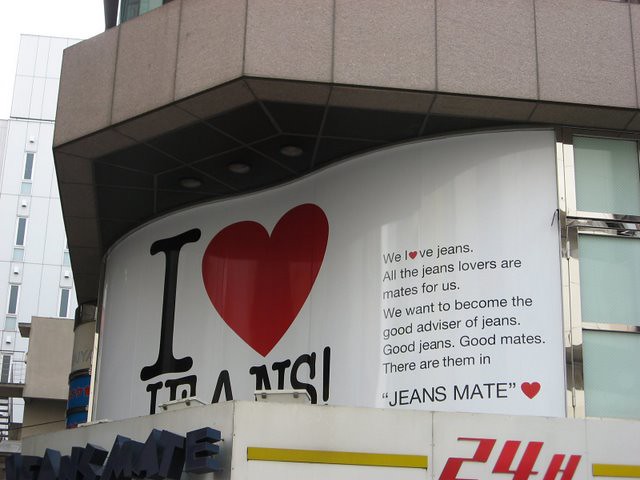In an urban setting, the image showcases the front of a building with a distinctive wavy white wall and an overhanging dark gray cement wall. Affixed to this wall is a large, eye-catching sign with a prominent white background. The sign features bold, black letters that spell out "I ♥ jeans," with a large red heart representing the word love. To the right of this main text, additional black lettering provides further context, reading, "We love jeans." Here, the O in "love" is creatively depicted as a red heart. Below, more text reads, "All the jeans lovers are mates for us. We want to become the good advisor of jeans, good jeans, good mates. There are them in jeans mate," followed by another red heart. Beneath the main sign, there's an additional red text element that reads "24H" with a horizontal red stripe, indicating the store operates 24 hours. The building also has a tan overhang above a window, which further solidifies its urban storefront presence.